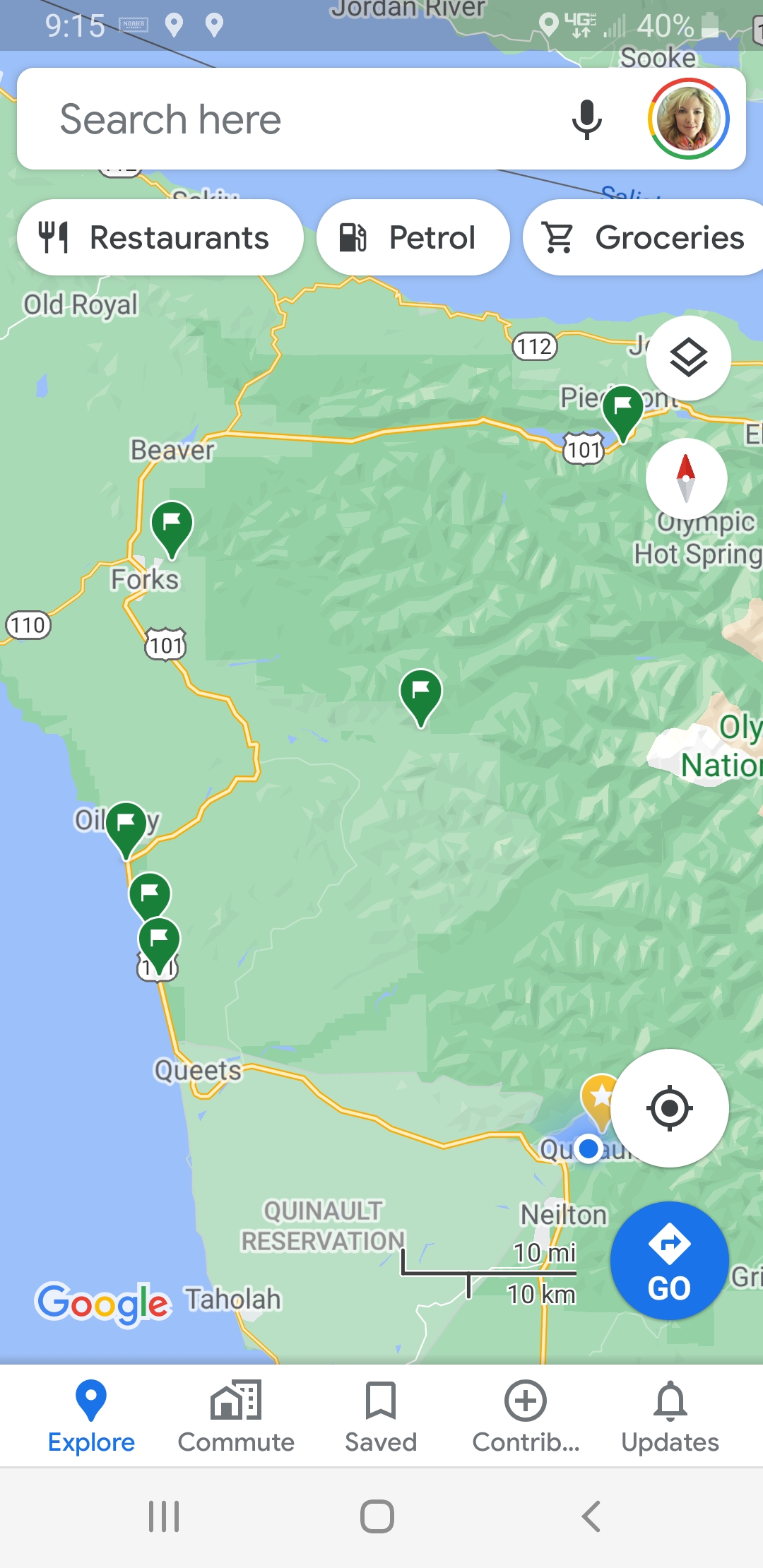This is an image captured from Google Maps. In the top left corner, the time "9:15" is clearly displayed. The top right corner features a small logo or possibly a user portrait. The prominent search bar in the center is accompanied by a microphone icon, symbolizing voice search functionality. At the bottom of the image, there's a section indicating the country, prominently displaying national flags. The interface elements and layout make it evident that this is a screenshot from a mobile or desktop version of Google Maps.